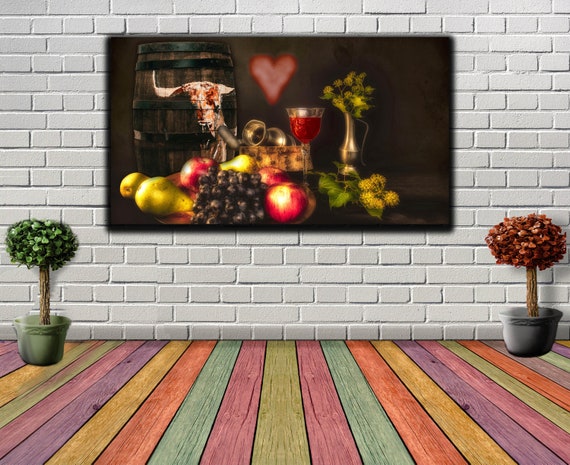This photorealistic, AI-generated image presents an intriguing room interior. The room's floor is covered in weathered, multicolored wooden planks, with hues ranging from yellow, orange, green, pink, and purple arranged in a random order. Dominating the top three quarters of the image is a white brick wall. Mounted on this wall is a large, visually compelling artwork with a dark brown background, prominently featuring a wooden wine barrel on the left side. The barrel displays an embossed image of a longhorn skull, giving it a rustic feel. In front of the barrel is a carefully arranged pile of fruits, including apples, grapes, and pears, alongside a wine glass and some flowers. Rising behind this still life scene is a distinctive pink heart. Flanking the painting, two potted plants add a touch of greenery: the plant on the left boasts green leaves, while the one on the right has red leaves. The image has a photoshopped quality, enhanced by the layered and somewhat incongruent placement of its elements.